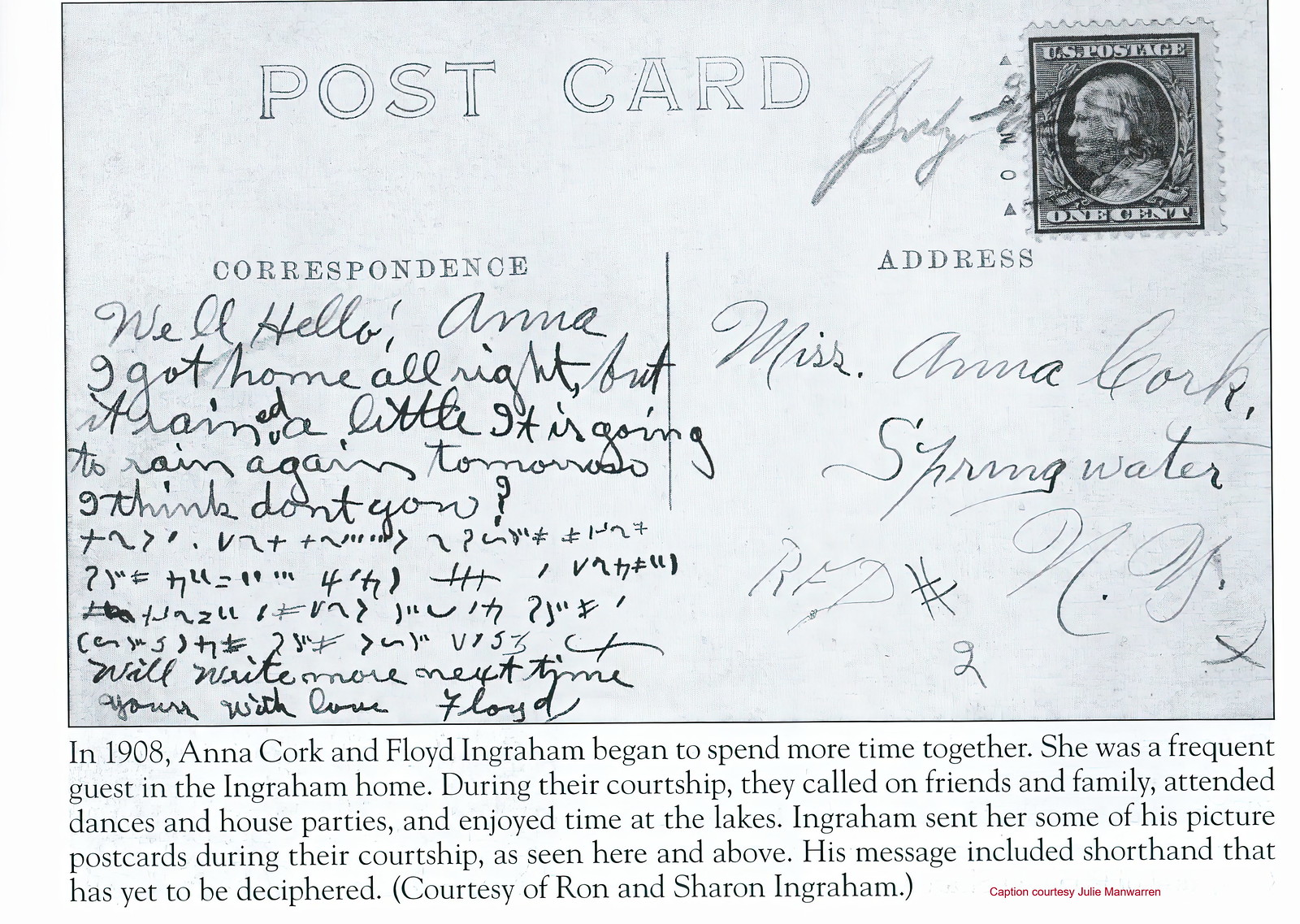This image depicts the back of a vintage, white postcard from 1908 with the word "POSTCARD" prominently displayed at the top in all capital letters. In the upper right corner, there is a 1-cent U.S. postage stamp with "July" handwritten nearby in cursive. Below the stamp, the areas labeled "Correspondence" and "Address" are also evident, separated by a centrally placed dividing line.

The "Correspondence" section contains a handwritten note in cursive, beginning with "Well, hello Anna," and indicating that the sender, presumably Floyd Ingram, got home safely but mentioned some rain. The message becomes increasingly difficult to decipher due to shorthand symbols towards the end, concluding with "With love, Floyd."

In the "Address" section, the recipient is listed as "Ms. Anna Cork, Springwater," but much of the writing here is scribbled and hard to make out.

Below the postcard image, a detailed historical context is provided, explaining that in 1908, Anna Cork and Floyd Ingram began to spend more time together, with Anna being a frequent guest at the Ingram home. During their courtship, they visited friends and family, attended dances and house parties, and enjoyed time at the lakes. Ingram sent Anna many picture postcards during this period, often including shorthand that is yet to be deciphered. The caption concludes with an attribution to Ron and Sharon Ingram for preserving this piece of history.

Finally, credit for the caption is given to Julie Merriman, noted in red font below the black-typed historical context.